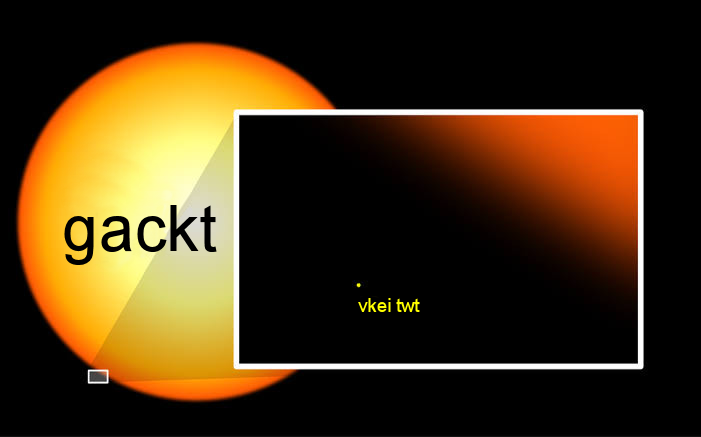The image is a digitally created diagram set against a pure black background. Dominating the left side is a large, yellow circular orb with a bright white center that transitions to a vivid yellow and then an orange outer edge. This suggests it may represent the sun or another celestial body. The orb features text reading "G-A-C-K-T" in black. Overlapping this orb on its right side is a white rectangular box, which appears to offer a zoomed-in view of the orb's edge. This smaller rectangle contains smaller text in yellow, "V-K-E-I-T-W-T," next to a small yellow dot below the orange section of the orb. The detailed color palette includes black, dark orange, light orange, yellow, and white, contributing to the depiction of some solar phenomenon or space-related imagery.